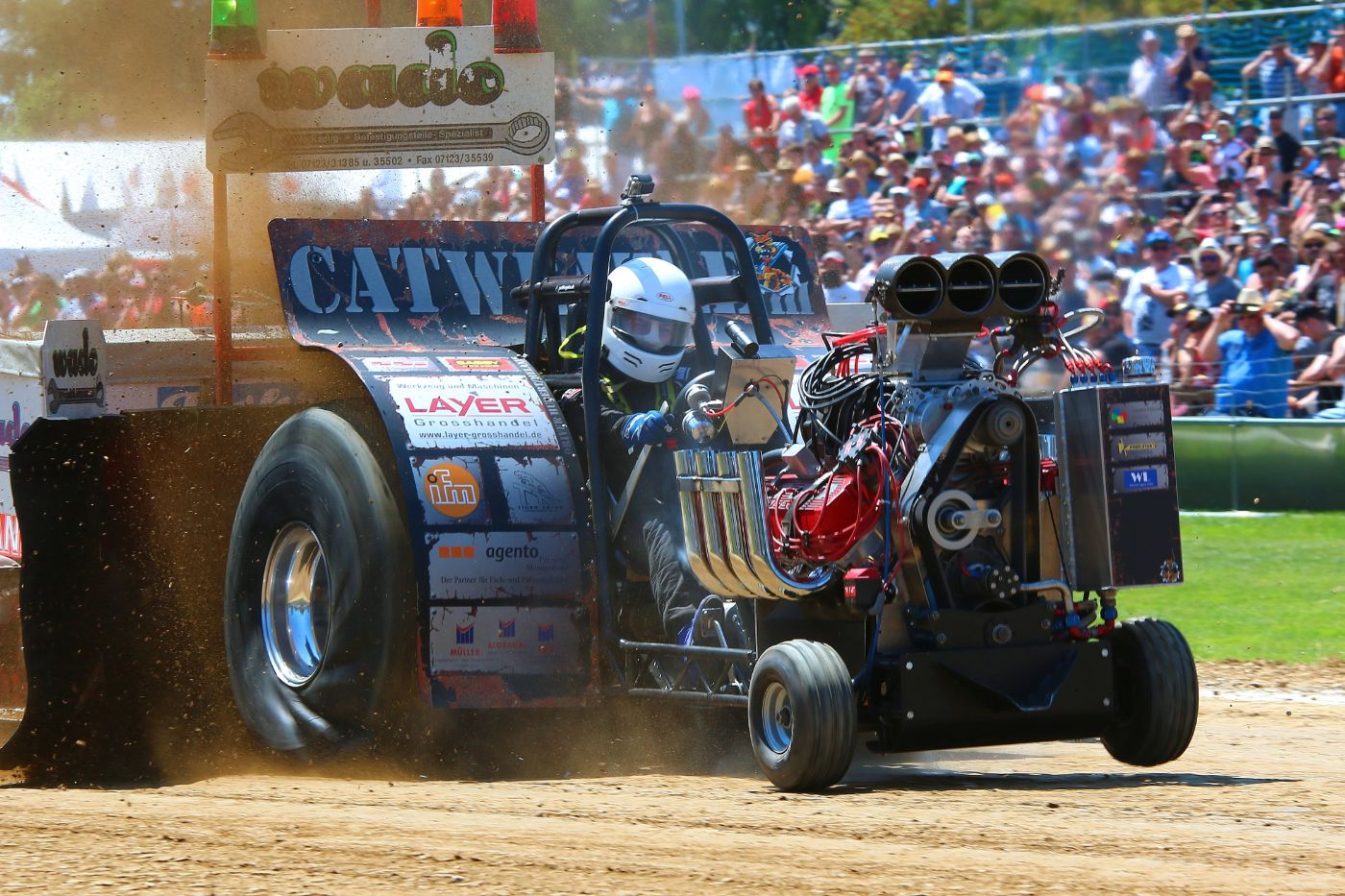This photograph captures a racing event taking place on a dirt track with a grandstand full of spectators in the background, many of whom are holding up cameras or binoculars. The focal point of the image is a highly unusual race car with a unique configuration: it has very large wheels in the back and very small wheels in the front, one of which is off the ground, indicating motion and speed. The car's engine is completely exposed, with four visible metal pipes protruding from it, and there are various sponsor stickers on its sides, including ones that read "Layer Gross Handle" with a website (www.layergrosshandle.de) and "Agento." The driver, dressed in a black suit, blue gloves, and a white helmet with a clear visor, is seated in an open cockpit secured with safety bars. Dirt is being kicked up by the tires, adding to the dynamic feel of the scene. The bright, sunny weather enhances the vividness of the image, highlighting the excitement and energy of the event.